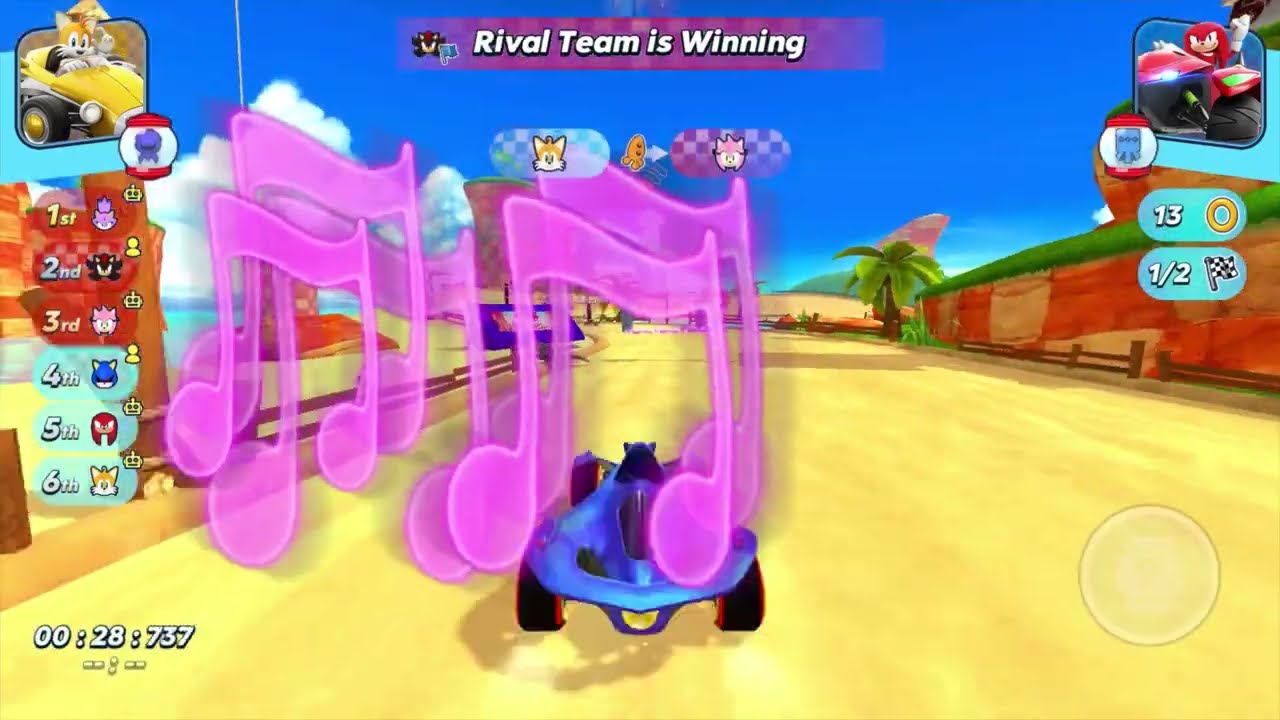The image is a vibrant, still shot from a child's or young adult's racing video game, possibly resembling a Sonic the Hedgehog or Mario Kart game, distinguished by its bold and varied colors, which include purplish pink, blue, yellow, gold, brown, green, light blue, black, white, orangish red, and orange. The main game screen features a central, small blue four-wheeled car driven by a character, surrounded by large, floating purple musical notes. The setting includes a dirt track lined with grass and hills, as well as a green palm tree, with additional buildings seen on the road's side. A bright blue sky filled with white clouds forms the backdrop. The game's status text, "Rival team is winning," is displayed prominently at the top center of the screen, contributing to the competitive atmosphere. A timer is located in the bottom left corner, and icons indicating the positions of other characters in yellow, red, and varied cars are shown on the left side, indicating the standings from first to sixth place. The image conjures an engaging and dynamic racing experience, imbued with musical elements making it both visually and interactively rich.